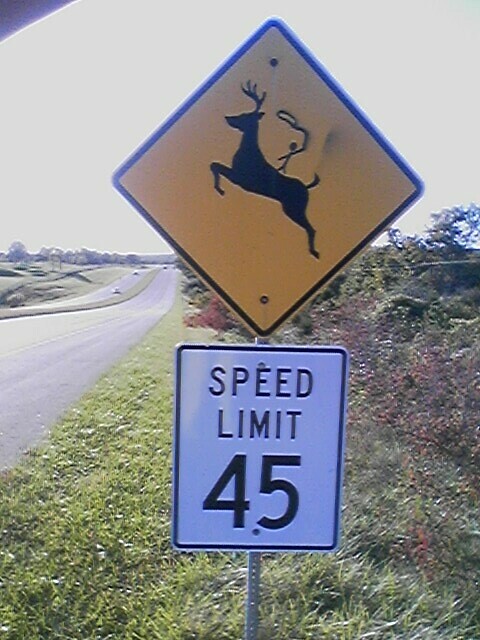This daytime photograph, though blurry and grainy, captures a detailed scene of a two-lane highway flanked by a green median. Positioned on the shoulder of the road, we face directly towards a metal pole adorned with two signs. The lower sign displays a speed limit of 45, while the upper sign warns of deer crossings with a yellow diamond-shape featuring a leaping deer graphic. Interestingly, a graffiti artist has added their own touch by painting a small stick figure riding the deer and holding a lasso. A smudge of paint appears next to the deer's tail. In the background, several cars can be seen traveling in both directions. The surroundings are lush with abundant greenery, and trees dot the distant landscape.